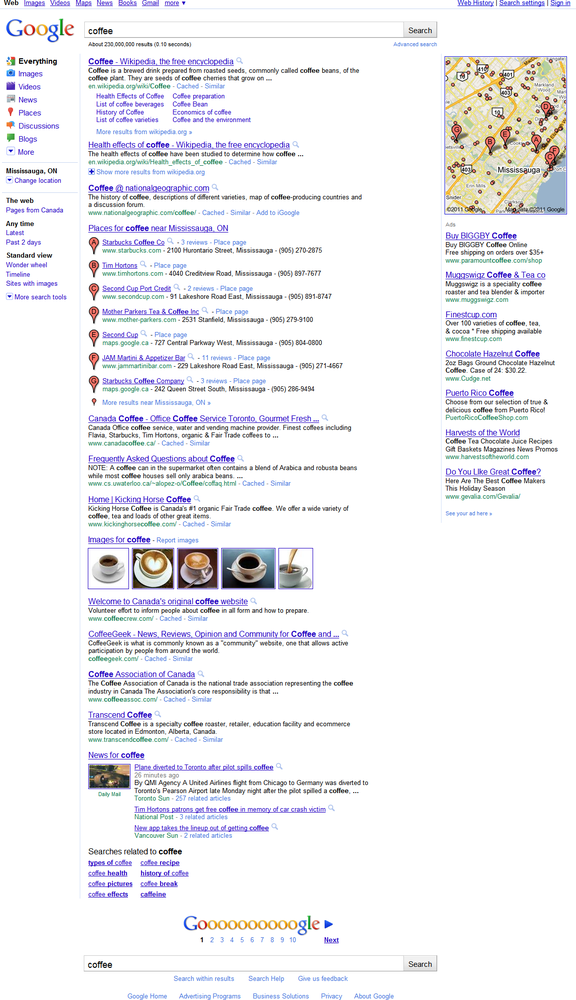Screenshot of Google Search Results for Coffee

In this detailed screenshot of Google search results for "coffee," we are presented with a densely packed and somewhat chaotic view, indicative of the depth and breadth of information available on this ubiquitous topic. At the top left, the familiar Google logo anchors the page, accompanied by a diverse menu bar offering various search categories: Everything, Images, Videos, News, Places, Discussions, Blogs, and more, suggesting a comprehensive search function.

The search has yielded an astronomical 230 million results, sprawling over at least 10 pages. Although it's unclear if the screenshot was captured on a tablet or another device, the interface is clear and functional. The user's location is set to Mississauga, Ontario, with an option available to change the geographic settings.

The primary search results begin with a prominent link to the Wikipedia page for "Coffee, the free encyclopedia." This is immediately followed by a page on the health effects of coffee. Next in line is an entry from National Geographic, highlighting coffee. The search results are supplemented with a series of Google map locations labeled from A to G, pinpointing local coffee spots around Mississauga.

The right column is dominated by a Google map featuring these marked locations, each with a corresponding link and brief description below the map. 

In the central panel, additional contexts about coffee in Canada appear alongside an assortment of images. These images predominantly consist of stock photos depicting various cups of coffee, some with cream, some without, reflecting the universal appeal and typical presentation of this beloved beverage.

Scrolling further reveals an endless array of links related to coffee, accentuating the exhaustive nature of this search. This extensive and content-rich screenshot encapsulates the quintessential Google search experience: boundless information, visually organized yet seemingly overwhelming due to its sheer volume.